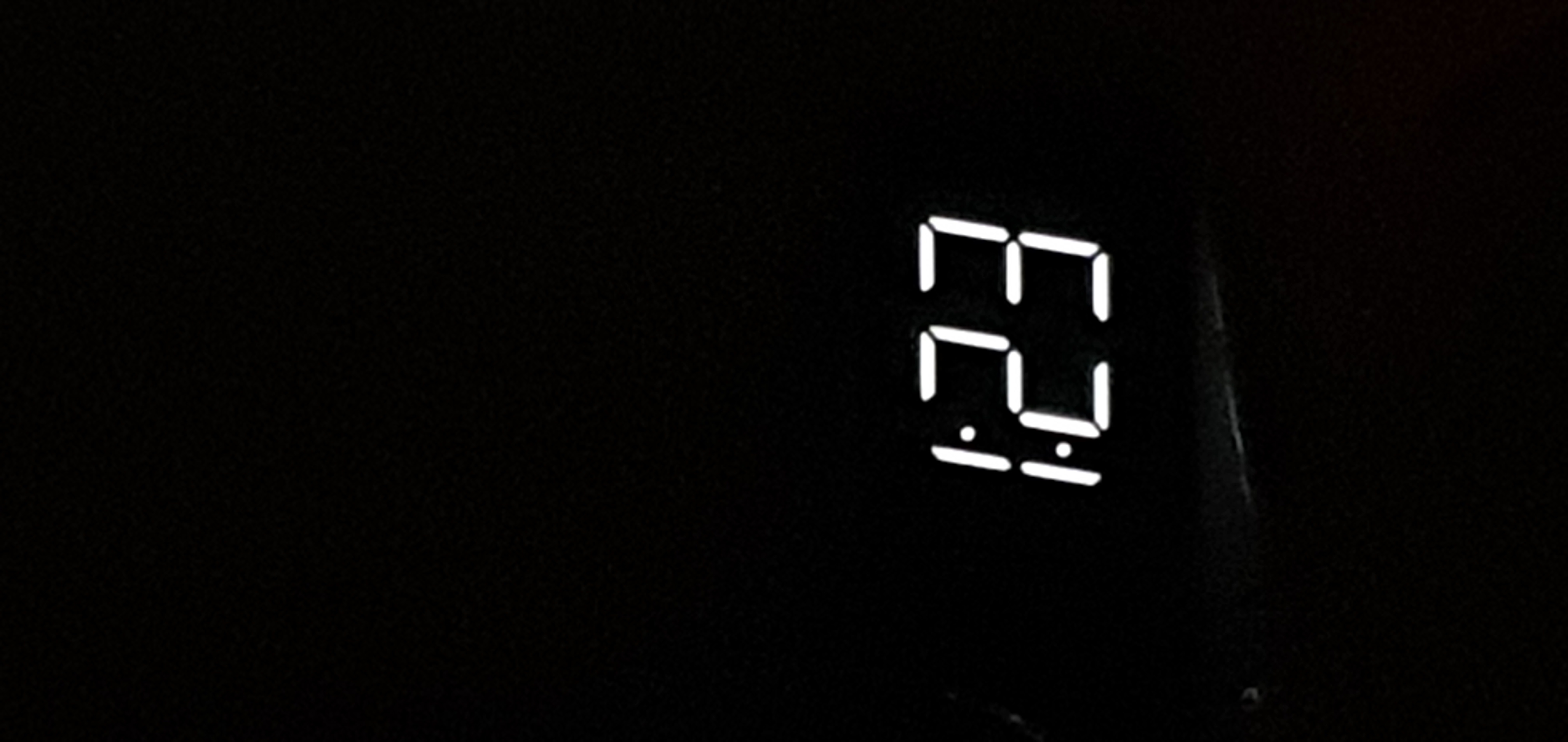The image depicts a sideways-oriented black-and-white photograph of a digital time display. The photograph, largely enveloped in darkness, prominently features the bright white numbers “1:23,” which might indicate the time as either 1:23 a.m. or p.m., though the surrounding darkness suggests it is taken at night. A faint reflection of the numbers appears in front of them, possibly on the edge of a tabletop or the surface beneath the clock. Additionally, there are a few small circular lights near the bottom right corner of the image. Aside from the illuminated numbers, no other elements are visible in the photograph, reinforcing the stark black background.